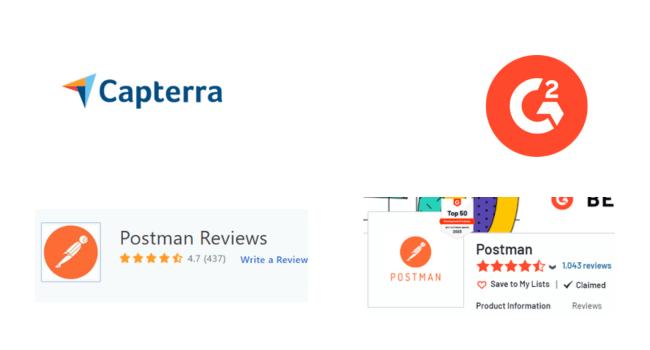The image is divided into four distinct sections, each showcasing logos and review snippets for the software tool Postman, sourced from two different review platforms: Capterra and G2. 

In the top left corner, the Capterra logo is prominently featured. The logo displays the word "Capterra" in blue text, accompanied by a stylized paper plane icon in blue, orange, and white.

Opposite this, in the top right corner, is the G2 logo. This logo consists of a bold red circle containing the letter "G," followed by a superscript "2" in white.

Beneath these logos, there's a section displaying snippets of reviews for Postman on Capterra. The Postman logo—a white postal horn silhouette set against an orange circle—appears on the left. Below it, the text "Postman Reviews" is shown in black. Adjacent to this are orange stars indicating the review rating of 4.7 out of 5, based on 437 reviews. To the far right of this section, there's a blue link labeled "Write a Review."

This detailed composition effectively merges brand logos, review ratings, and platform details to provide a comprehensive overview of Postman's reviewed performance on Capterra and G2.